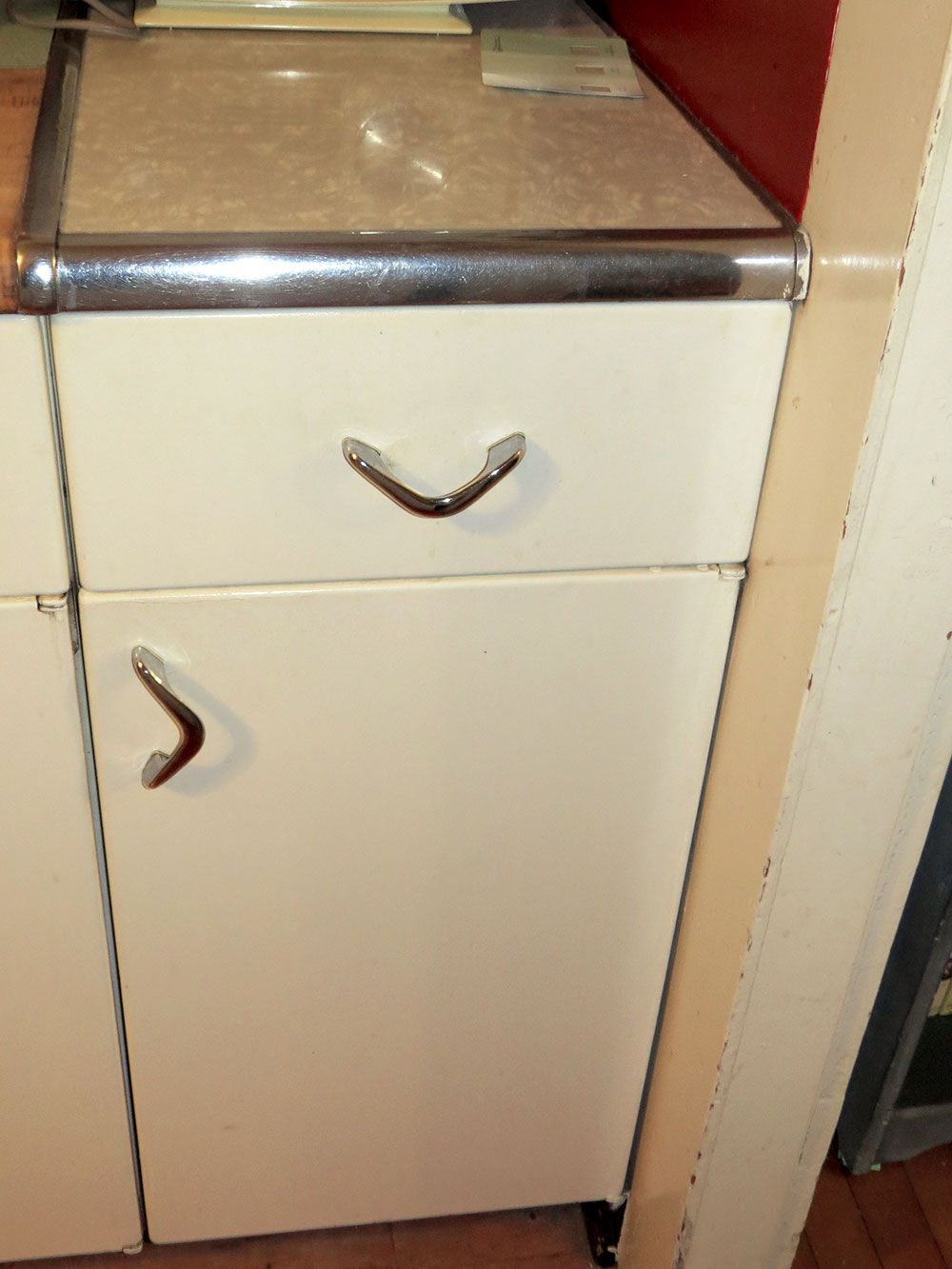This image features the bottom part of a vintage kitchen cabinet, likely from the 1950s or 1960s. The cream-colored cabinet, made of metal, has two V-shaped silver handles: one on a pull-out drawer positioned above and another on an elongated door below. A distinctive silver strip separates the brown laminate countertop, which mimics marble and is framed by a dark brown trim. Resting in the top right-hand corner of the countertop is a piece of white paper. To the right of the cabinet, there is a glimpse of a red wall connected to a white portion, and along the right side, a white trim can be seen. At the bottom edge of the image, there is a thin line of wood flooring visible. Overall, the setup exhibits a nostalgic, mid-century kitchen aesthetic.